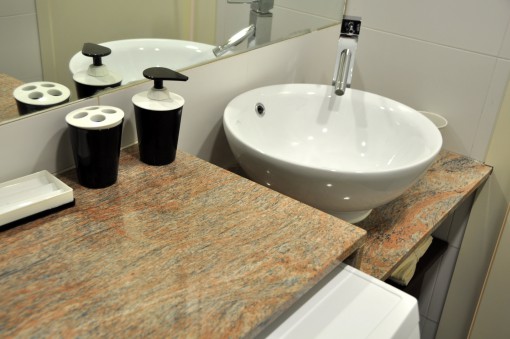The image portrays a well-lit bathroom captured from the position of the commode. In the lower portion of the photograph, part of the flush box is visible. Positioned above it is a granite countertop that extends across the scene. This countertop features several items: prominently, an empty soap bar tray, and to its right, a black cup with a white lid featuring four slots intended for toothbrushes, which are currently vacant.

Further to the right, another black cup is situated next to a matching black and white soap dispenser. A continuation of the granite countertop accommodates a small, pristine white bathroom sink. The sink is accompanied by a sleek, stainless steel faucet with a matching handle incorporating both black and steel elements.

Beneath the sink, a garbage bin can be seen, equipped with garbage liners. Adjacent to the sink sits a white cup, though its contents are not visible. The setup reflects a minimalist and monochromatic theme, emphasizing functionality and cleanliness.